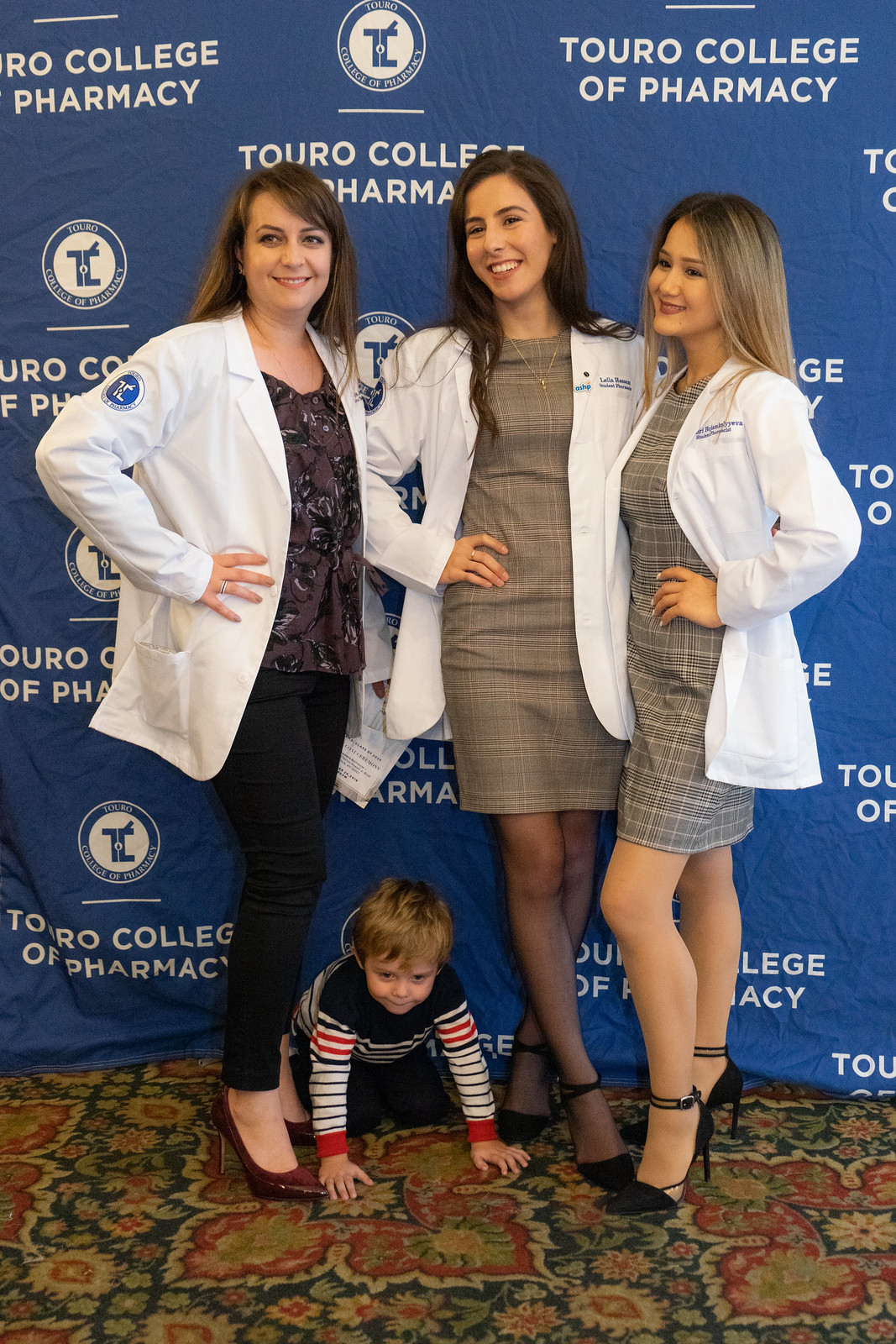In this image, three women stand side by side in front of a blue banner that reads "Touro College of Pharmacy" in white text. The woman on the far left is a white female with brown hair. She wears a white lab coat over a black and purple floral blouse, paired with black pants and burgundy high heels. Next to her, a little boy, around three years old, crawls on the ground. He has light brown or reddish hair and is dressed in a black long-sleeved shirt with white and red stripes. The woman in the middle, also a white female with dark hair, wears a white lab coat over a gray plaid dress and black high heels. The woman on the far right appears to be Asian with light brown hair, dressed similarly in a white lab coat over a gray plaid dress and black high heels. The carpet beneath them features a floral pattern in green and red hues.